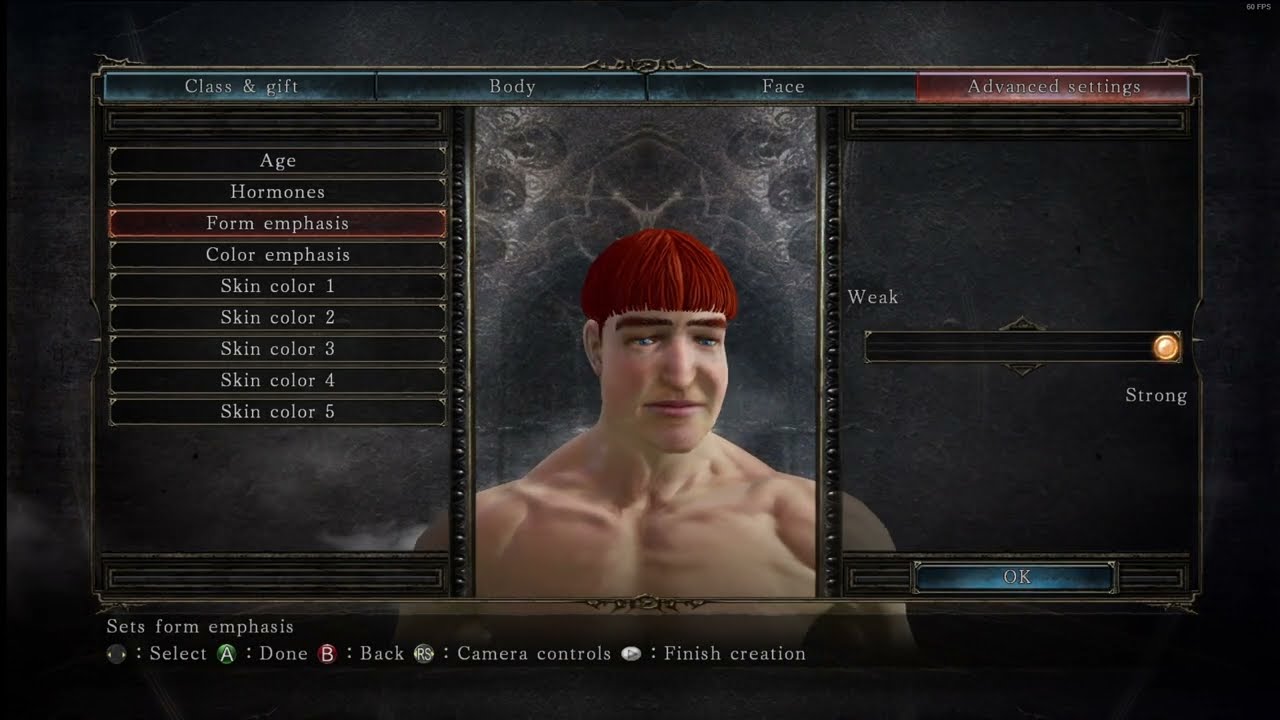The image is a screenshot of a character creation screen from a video game, shown within a horizontal rectangle with a dark gray or black background. The central focus is on a vertical rectangle depicting a muscular male avatar with pale skin, short red hair with bangs, thick reddish eyebrows, and light blue eyes. The avatar is viewed from the chest up and appears shirtless, with heavy sinewy muscles prominent on his chest and shoulders. A faint, indistinct emblem can be seen on the wall behind him.

Across the top of the screen, a horizontal bar is divided into segments labeled "Class and Gift", "Body", "Face", and a glowing red section labeled "Advanced Settings". Below "Class and Gift" on the left side, there are several horizontal buttons with white text on a black background, listed from top to bottom as: "Age", "Hormones", "Form Emphasis" (highlighted in red), "Color Emphasis", "Skin Color 1", "Skin Color 2", "Skin Color 3", "Skin Color 4", and "Skin Color 5".

On the right side of the screen, a vertical bar with white text indicators shows "Weak" at the top left and "Strong" at the bottom right. A yellow circle is positioned near the "Strong" label, indicating the avatar's current strength level. Below this, a blue button labeled "OK" is visible.

At the bottom of the image, additional controls are displayed with the text: "Sets Form Emphasis". There are icons and text labels stating "Select", "Done", "Back", "Camera Controls", and "Finish Creation".